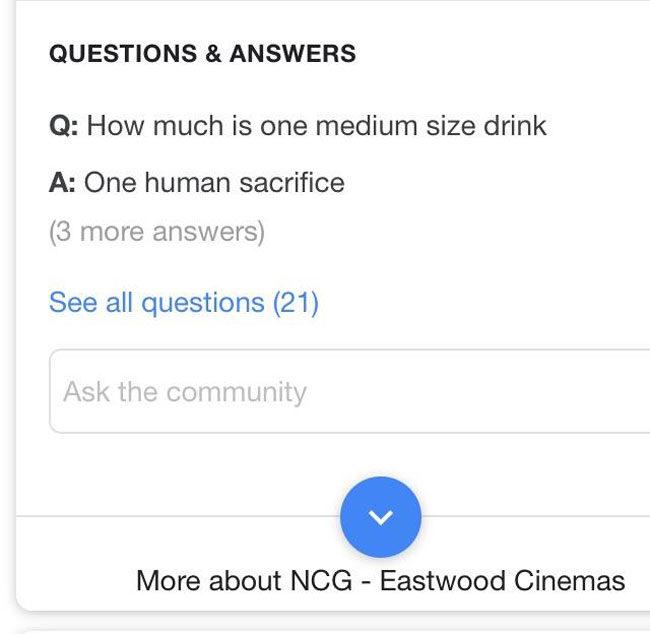The image features a clean white background outlined in light blue. At the top, in bold letters, it says "Questions and Answers." Below this heading, a question is presented: "Q: How much is one medium-sized drink?" with a humorous answer provided: "A: One human sacrifice," followed by parentheses indicating there are three more answers. Just beneath, a clickable link in blue text invites viewers to "See all questions," noting there are 21 in total.

In the middle of the image, there's a prominent box labeled "Ask the Community," designed for users to pose their own inquiries. At the bottom, separated by a dividing line, there's a large blue circle featuring a white checkmark. Adjacent to this emblem, it reads "More about NCG Eastwood Cinemas," offering further information about the cinema. The image is designed to be functional and interactive, guiding users through a Q&A section for a cinema's offerings.